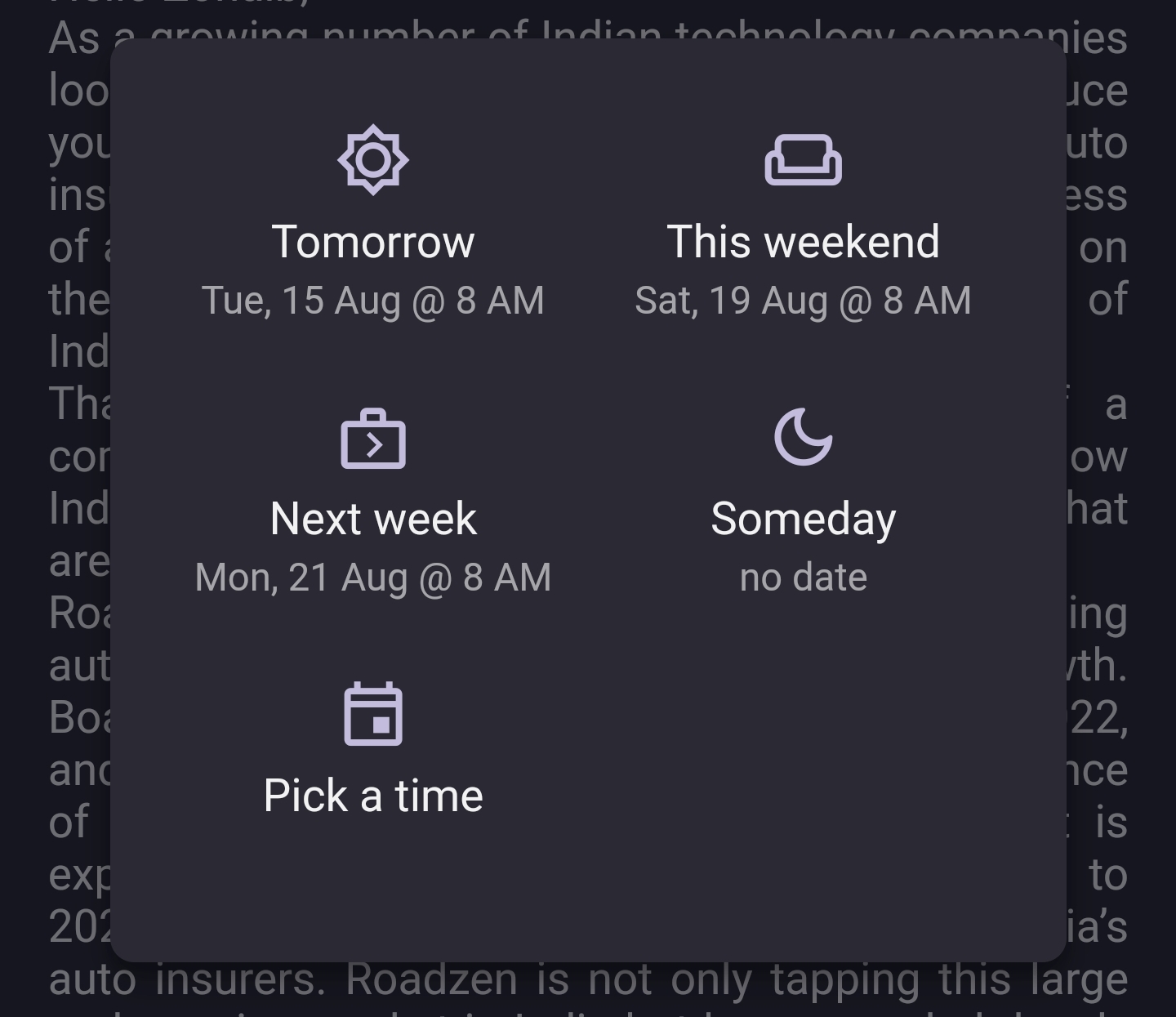This image depicts a screenshot from a mobile app's calendar interface. The background is entirely black with white text. Overlaying the background is a large, dark grey, opaque box that occupies most of the screen. This grey box also features white text and various white icons.

Within this box, there are five distinct entries:

1. The first entry, located on the left side, reads "Tomorrow, Tuesday, 15 August at 8am." 
2. Positioned underneath, the second entry states "Next week, Monday, 21 August at 8am," accompanied by a briefcase icon.
3. Further below is the third entry labeled "Pick a time," highlighted by a calendar icon.
4. On the right side of the box, the fourth entry says "This weekend, Saturday, 19 August at 8am," and it is marked with a couch icon.
5. Finally, at the bottom, the fifth entry reads "Someday, no date," distinguished by a crescent moon icon.